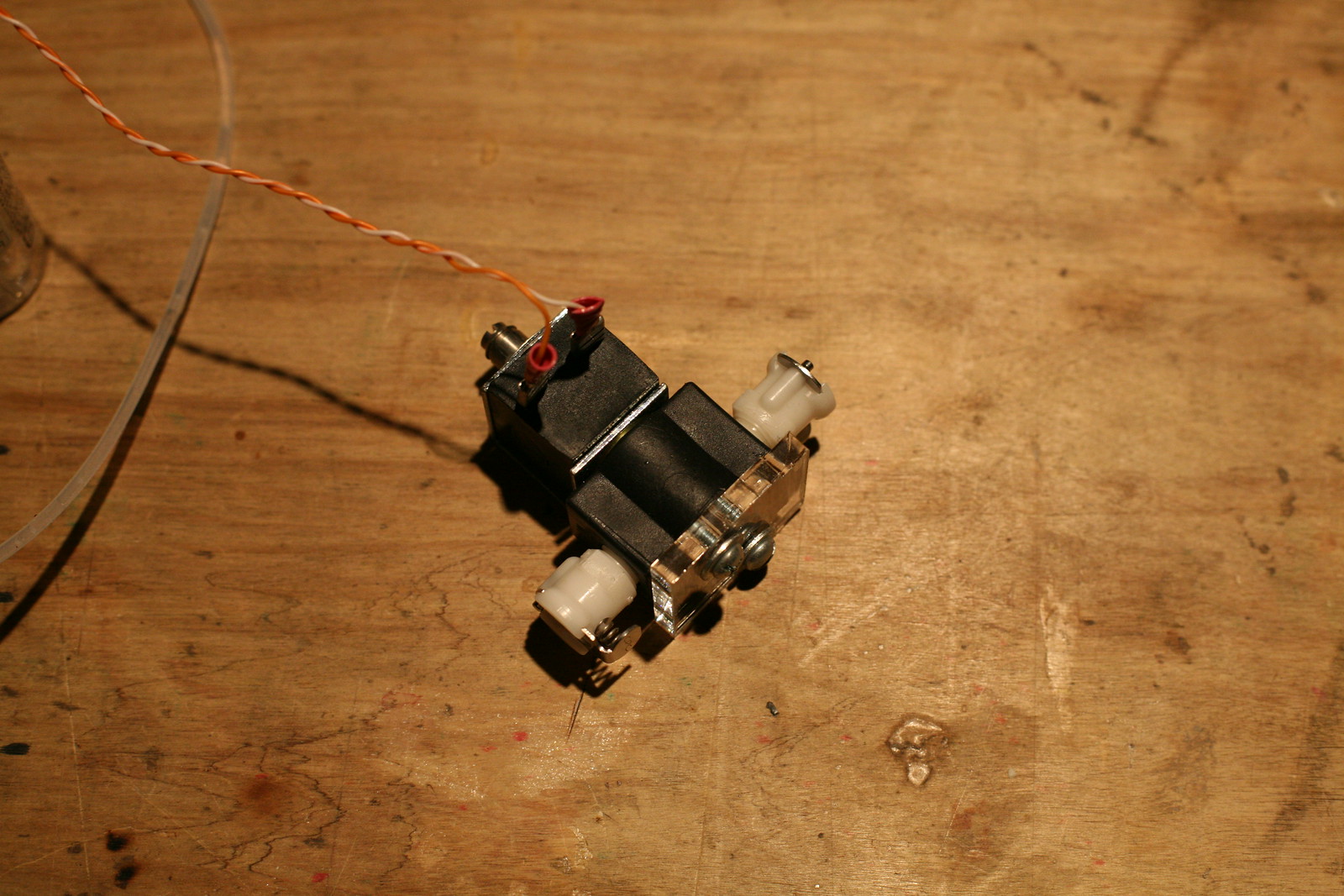The image depicts a complex electronic device placed at the center of a well-used wooden work table, which shows signs of glue stains, discolorations, and colored pencil or pen marks. The device, somewhat resembling an old-fashioned camera, is seen from above, making it challenging to precisely identify. However, it appears to involve a black main body with attached components. There are two distinct wires—one red and one white—that originate from two red holes in the device and intertwine as they head towards the top left-hand corner of the image. Alongside these wires, there is an orange wire accompanying them. On the left side of the black body, a phone line runs underneath the intertwined wires. The device also includes white plastic components with metal pieces protruding from both sides, which are connected to the black body. At the bottom part of the device, copper-colored metal and steel sections with metallic domes are visible. To the right, the device has a clear mirrored component. The entire setup rests on a piece of plywood. Some speculate that the device might be a large solenoid or consist of multiple solenoids, possibly including motors or latching mechanisms.